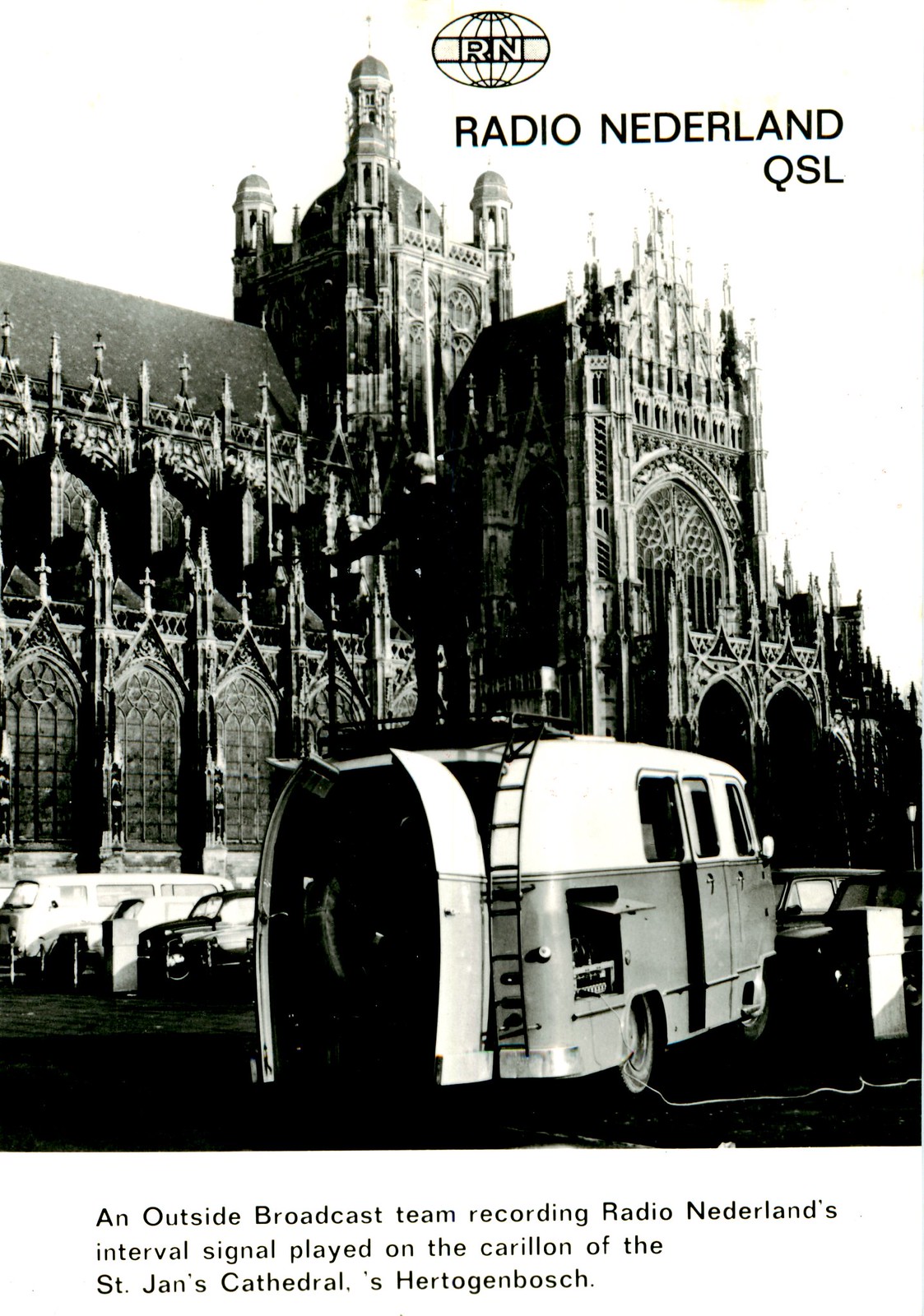This black-and-white photograph captures an intricate scene centered around the St. Jan's Cathedral in Hertogenbosch. Dominating the top three-fourths of the image, the ornate cathedral with its grand spires serves as a majestic backdrop. Below, centrally positioned towards the bottom of the image, a broadcast van with its back doors open is prominently featured, alongside other vehicles arranged in a parking lot to the left. A cord runs from the main vehicle, indicating it's being used by an outside broadcast team. The text in black uppercase letters reads "Radio Nederland QSL" and explains the scene: "An outside broadcast team recording Radio Nederland's interval signal played on the carillon of St. Jan's Cathedral, Hertogenbosch." The photograph, marked by varying shades of gray, underscores the historical and technical significance of the moment captured.